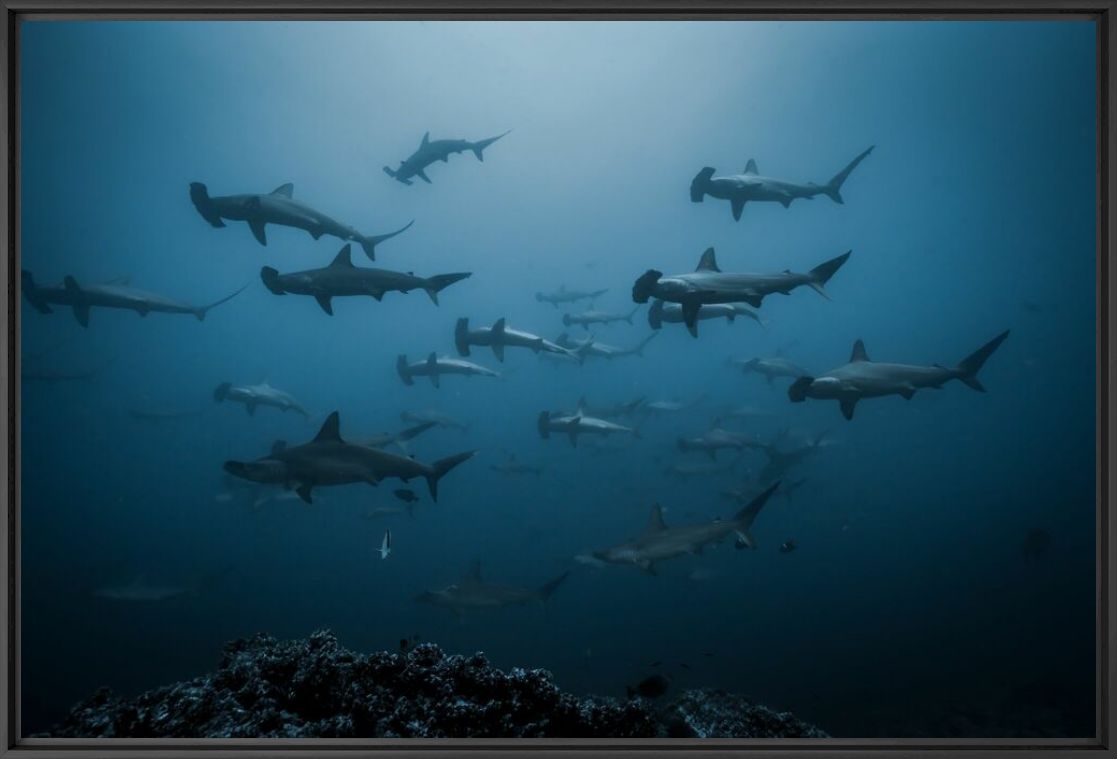The photograph captures a dark, underwater scene, almost on the ocean floor, where a large school of hammerhead sharks is swimming to the left. The dark tones of blue, black, gray, and white enhance the cold and slightly deep underwater atmosphere, indicating minimal sunlight penetration. There is some coral reef visible at the bottom, particularly on the bottom-left side. While numerous hammerhead sharks, with their distinctive hammer-shaped heads, dominate the scene—numbering into the dozens with some estimates suggesting as many as thirty—there are also a few other species, likely smaller nurse sharks and unidentified fish, adding to the bustling marine life. The image has a gradient background of blue and is detailed and professionally shot using an underwater camera, showcasing the varied shades and shadows that make the scene both dynamic and somewhat shadowy. Overall, the photograph is a vivid depiction of marine biodiversity, emphasizing the hammerhead sharks prominently.